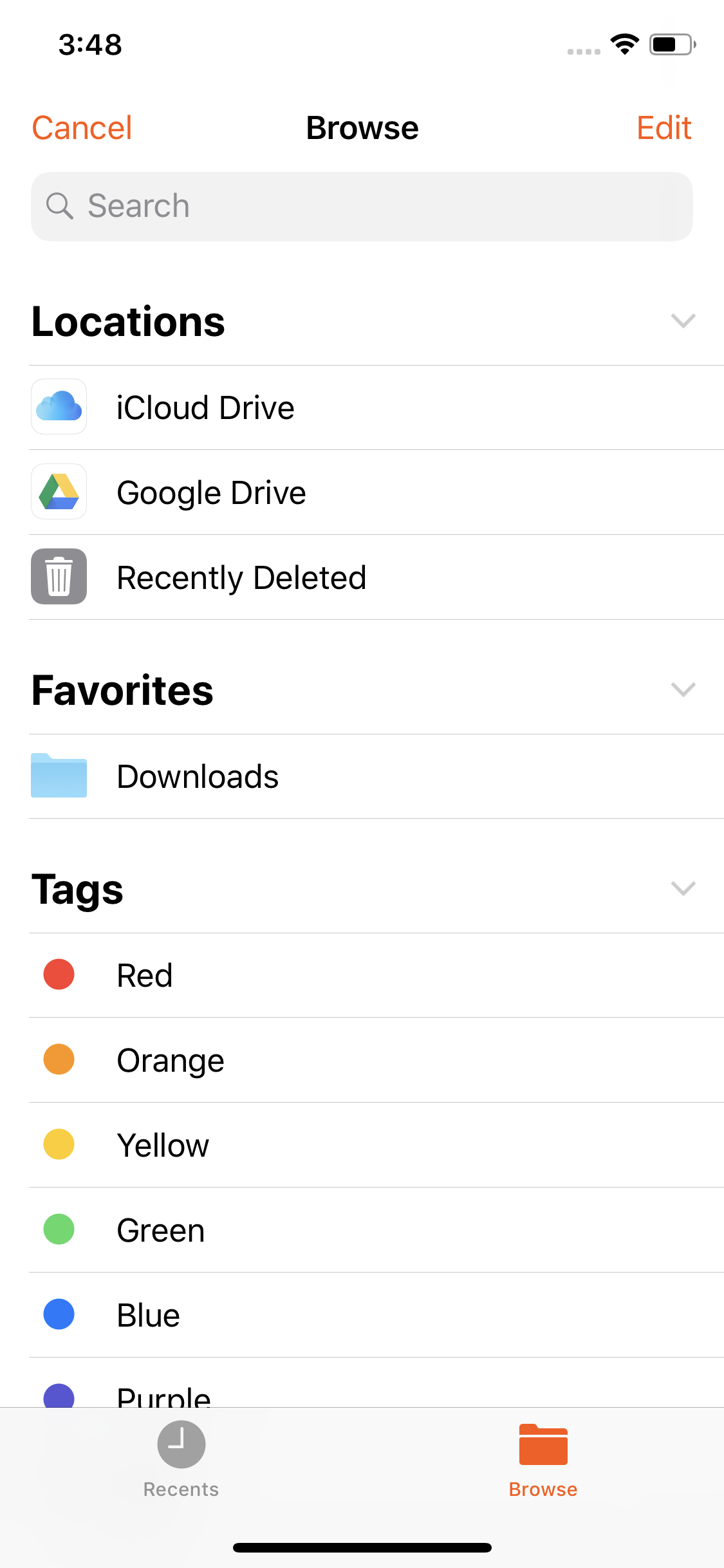The screenshot features the user interface of a file management application displaying the "Browse" section. At the very top, there are "Cancel" and "Edit" options. Beneath them, a search bar is present, characterized by a gray background, a magnifying glass icon, and the word "Search" in dark gray text.

The main section is divided into categories, with "Locations" listing various cloud services and recently deleted items. In this section:
- "iCloud Drive" is represented by a blue cloud icon.
- "Google Drive" is signified by the iconic green, yellow, and blue triangle.
- "Recently Deleted" features a gray square with a white trashcan icon.
  
Under "Favorites," there's an entry for "Downloads," indicated by a blue file folder icon.

The "Tags" section displays a series of color-coordinated circles:
- Red,
- Orange,
- Yellow,
- Green,
- Blue,
- Purple.

At the bottom of the screen, the "Recents" section is marked by a gray circle with a white clock icon and the word "Recents" in gray.

Lastly, as part of the navigation, the "Browse" category is highlighted with an orange file folder icon.